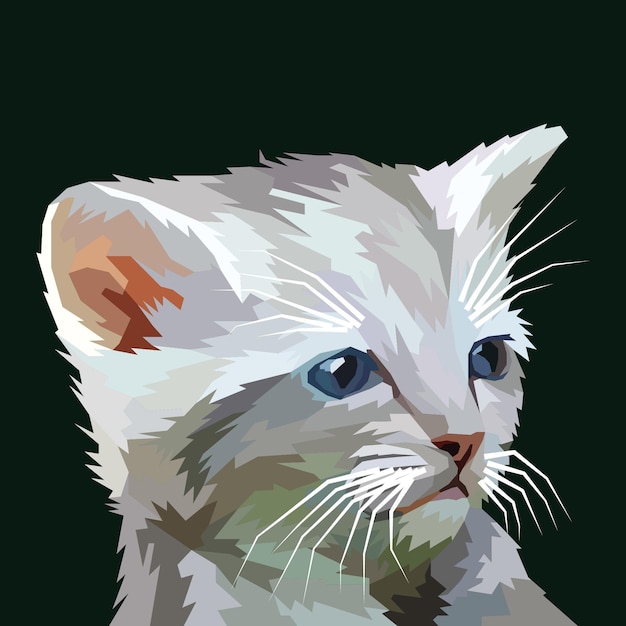This is a digitally created, cartoonish graphic of a white cat with shades of light and dark gray fur, giving the impression of shadowed areas. The cat is shown from the shoulders up, positioned against a solid black background, looking off to the right. It boasts striking blue eyes with black pupils, long white whiskers on its cheeks, and additional whisker strands where its eyebrows would be. The interior of its ears displays natural hues of brown and pink. The cat's fur is notably lighter on the top of its head and its cheeks, transitioning to a darker gray at the bottom, likely due to lighting effects to simulate shadows. The art style eschews outlines, relying solely on color variations to define the cat's features, giving it a seamless, painted appearance.